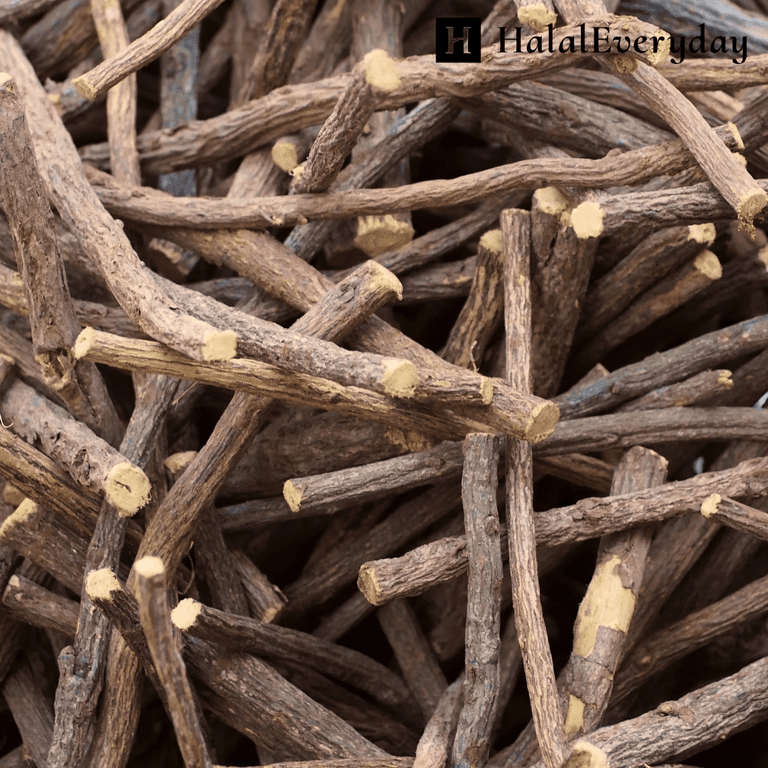This detailed close-up image showcases a disordered pile of slender twigs or branches, each about 3-4 inches long and varying in diameter from half an inch to ten centimeters. These twigs, retaining their natural bark, have lighter yellowish-brown ends where they have been freshly cut, giving them an appearance evocative of either licorice sticks or small cut branches. The image is tight and focused, intensifying the texture and disarray of the pile, which some might compare to the intricate structure of a beaver dam. 

In the upper right-hand corner of the photo, a black square with a cutout letter "H" stands out. Beside this logo, the phrase "Halal Every Day" is inscribed in elegant black lettering, adding a modern and slightly mysterious element to the otherwise rustic and natural scene.